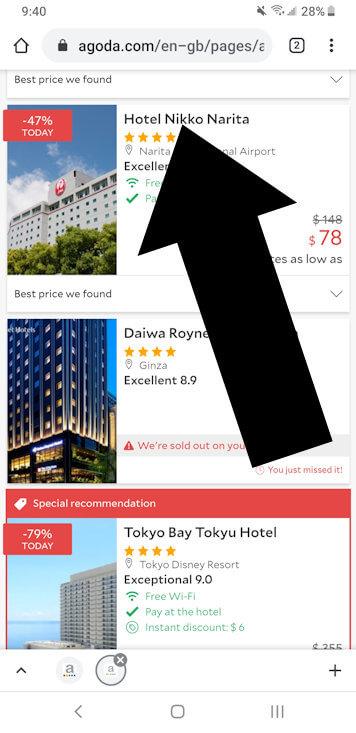This image is a cropped and edited screenshot from a booking website for accommodations. A large black arrow has been added, pointing directly towards the top entry on the list, which is Hotel Nico Narita. The arrow is angled to the right but clearly highlights Hotel Nico Narita. On the left side of the screenshot, it shows a notification that reads "down 47% today" in the top left corner. To the right, the hotel name "Hotel Nico Narita" is visible. Beneath it, the visible part of the description includes the rating "excellent" and various amenities, though part of the information is obscured by the black arrow. The price per night is listed as $78. At the bottom of the screenshot, another listing has a red border on the top with the label "special recommendation."